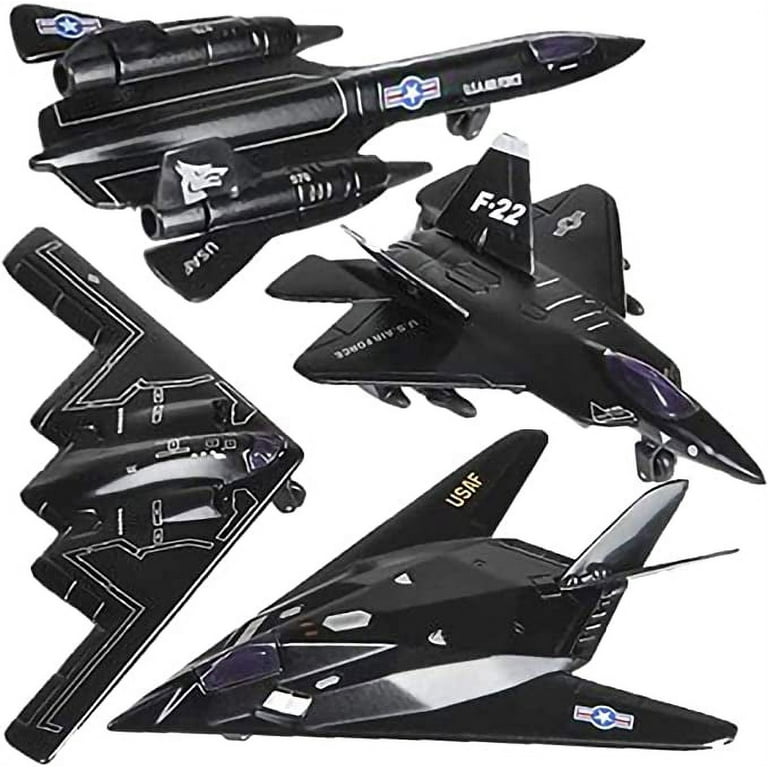This image features four sleek, black model aircraft displayed against a white background, each with distinctive characteristics and markings, predominantly associated with the United States Air Force (USAF). 

At the top is a cylindrical jet with a dragon head design and a pair of large rockets on its wings. It bears the USAF insignia with a white star encircled in blue, flanked by red and white stripes.

Below this, to the right, is a slightly shorter jet with a long, slender nose and triangular body. It has distinctive pointed wings extending from either side and is marked "F-22" and "US Air Force" in bold white letters.

To the left of the F-22 is a jet with a triangle-shaped body and a cut-out W design on its back half. It features long, skinny wings on the sides, adorned with white accents and a unique design, though it lacks specific text inscriptions.

At the bottom right is another triangle-shaped aircraft tapering into a V at the rear, with a long, slender fin extending from the top. This model also displays the "USAF" marking. All the models shine with a dark metallic finish and share white accents, emphasizing their coherent aesthetic and connection to the Air Force.